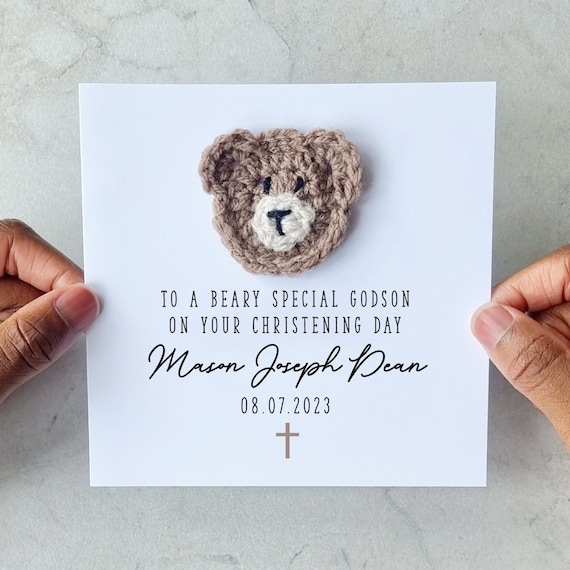A photograph features a christening announcement card held by well-groomed African-American woman's hands, visible only by the thumb and forefinger on either side. The backdrop is a grayish-white marbled wall. The card itself is a small, simple white piece of cardstock adorned with a sweet, handcrafted, crocheted teddy bear head—brown with a white muzzle, black eyes, and a black nose. The card reads, "To a BEARY special godson on your christening day," with the name "Mason Joseph Dean" written in elegant cursive, followed by the date "08-07-2023" and a Christian cross emblem. This charming, partially handmade card highlights the personalized and heartfelt nature of the celebration.